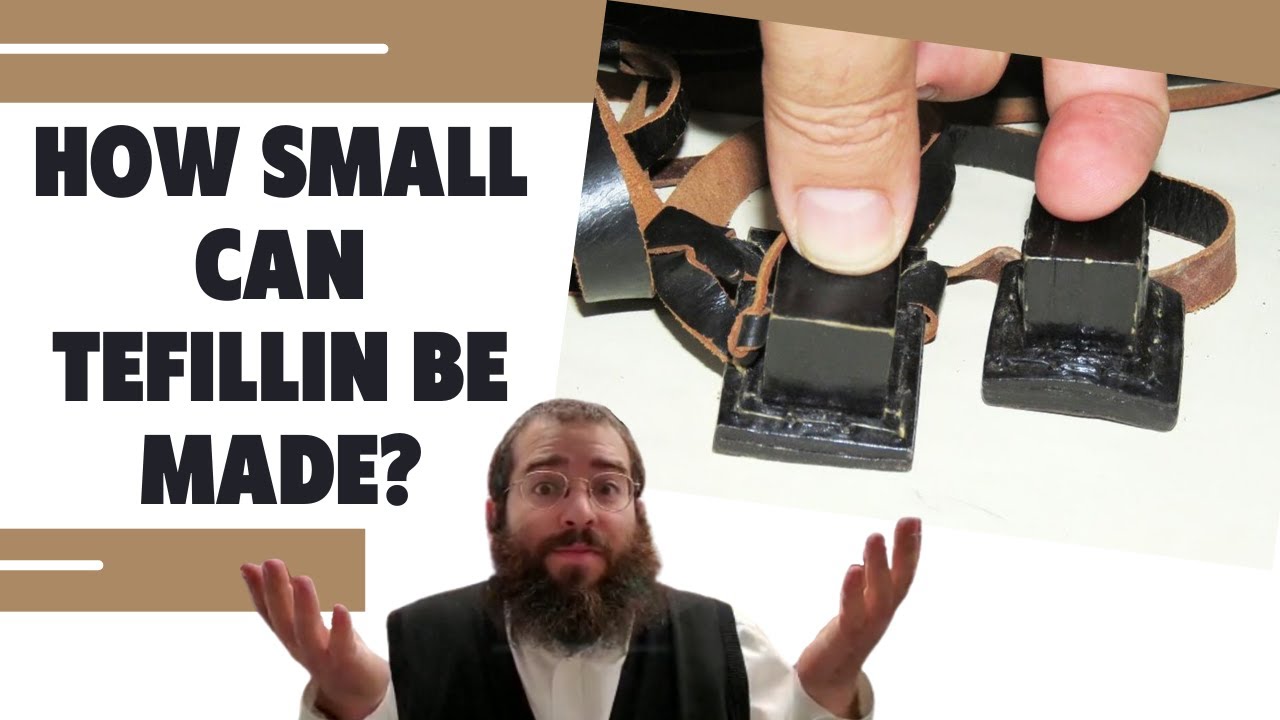The image features a man positioned centrally at the bottom, showing his head and chest while holding his hands up to his sides, as if asking, "What happened?" He has a neatly trimmed beard and short hair, and he wears a black vest over a white shirt. The background is predominantly white, with two light brown stripes—one at the top and another beneath a section of text. 

The text, located in the upper left quadrant, reads in large black letters: "How small can Teflon be made?" To the right, a close-up shows a person's thumb and fingers holding two small black blocks, each equipped with black and brown leather straps. These blocks, potentially made of Teflon, have a possible connection to Jewish ritual items known as Tefillin, given the context of the leather straps. The upper right quadrant's white background mirrors the rest.